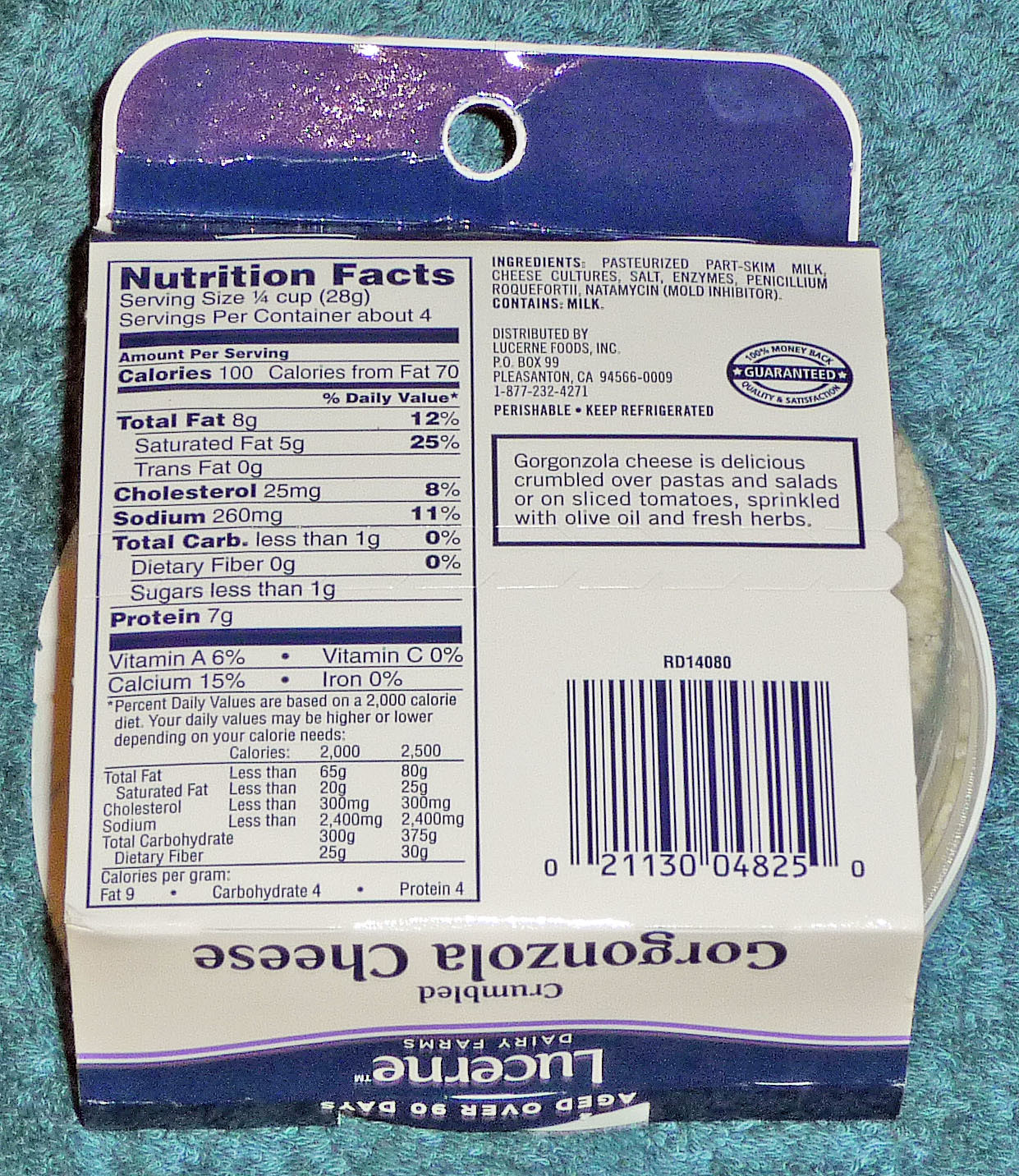The image showcases the backside of a package of crumbled Gorgonzola cheese by Lucerne Dairy Farms. The package is positioned upside down on what appears to be a brushed blue tabletop. The top of the package features a blue section with a hole for hanging on a rack, bordered by white trim. The central portion is white with blue text, including detailed nutritional information. Each serving of the cheese contains 100 calories, 8 grams of fat, 25 milligrams of cholesterol, and 260 milligrams of sodium, with the container offering four servings.

Key product descriptions indicate that Gorgonzola cheese is delicious when crumbled over pastas, salads, or sliced tomatoes, and sprinkled with olive oil and fresh herbs. The package mentions that the cheese is aged over 90 days and includes a blue barcode in the bottom right corner. The left side of the package features the nutrition facts, while the top right houses the ingredients list and the distributor's information: Lucerne Foods from Pleasanton, California. There's also a 100% money-back guarantee and a note stressing that the cheese is perishable and must be kept refrigerated. Ingredients include pasteurized part-skim milk, cheese culture, salt, enzymes, Penicillium Roqueforth, and natamycin as a mold inhibitor.